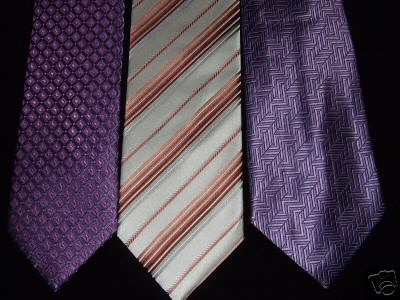The image showcases three distinctive neckties arranged in a row on a black background. Prominently lit, the ties are the main focus, and each offers a unique design. On the left, the first tie is a deep violet-purple featuring a diamond-shaped pattern with small white spots in the center of each diamond. The middle tie stands out with its vintage look, sporting diagonal stripes in shades of orange, red, and white, reminiscent of styles from the 1970s. On the right, the final tie is a slightly lighter purple with a complex, maze-like design that conveys a textured, almost scratchy material. Notably, a watermark in the bottom right corner of the image resembles the transparent icon of an old-fashioned analog camera, possibly indicating the image was hosted on the picture-sharing site PhotoBucket.